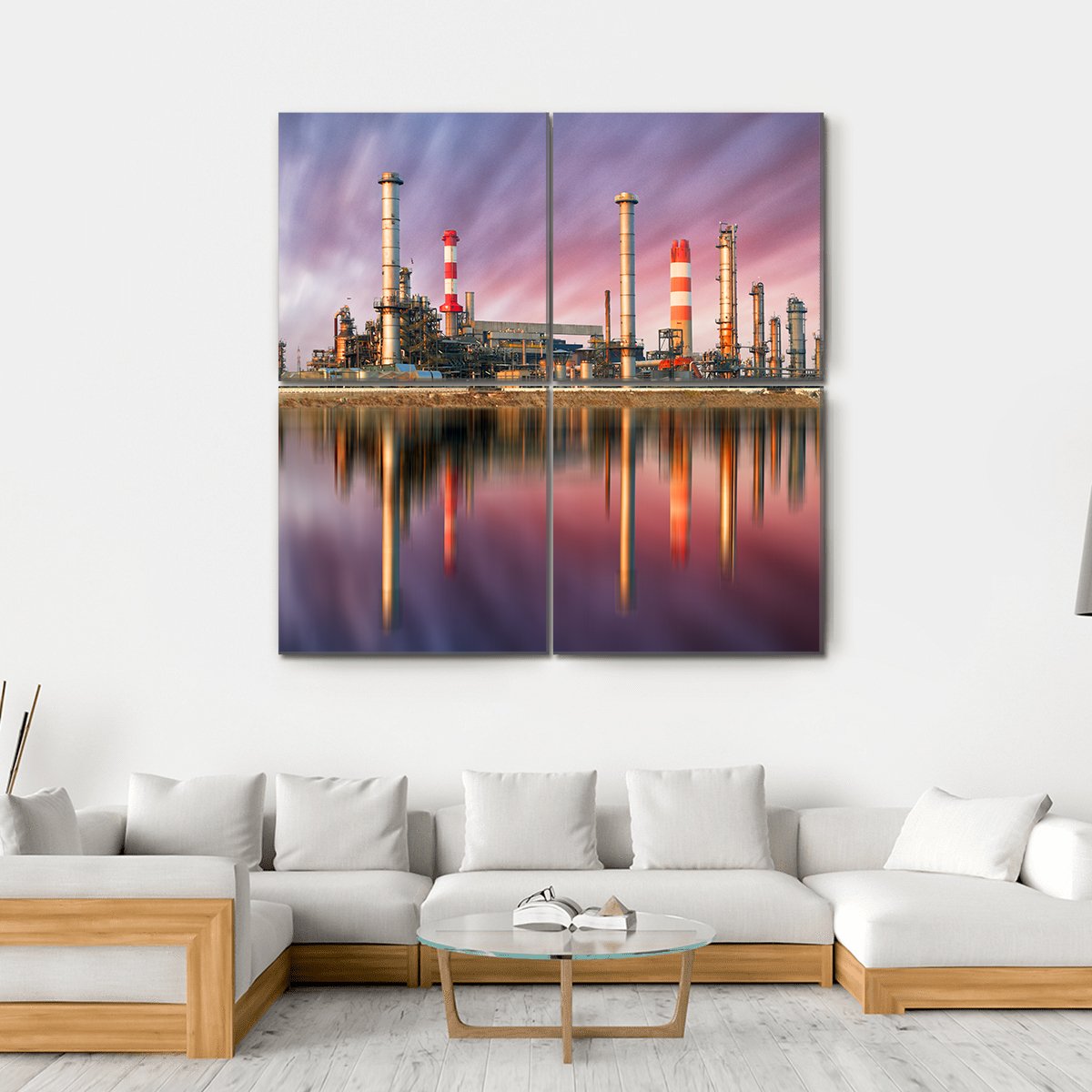The image showcases a pristine white living room with a clean, modern aesthetic. The focal point is a large white couch featuring a wood platform base and armrests, adorned with six plush throw pillows. This spacious couch, capable of seating six to seven people, is complemented by a sleek round coffee table with a glass top and a wooden base, which supports an open book in front of it. The room has a light grey wood plank floor that enhances the airy and bright ambiance. Above the couch hangs a striking four-piece artwork, assembled in a 2x2 grid. The artwork depicts industrial refinery machinery with tall, colorful silos and metal cylinders, set against a coastal backdrop where the shoreline and structures are elegantly reflected in the water. The sky in the artwork is a captivating blend of purple and pink hues, adding a dramatic touch to the room's décor.